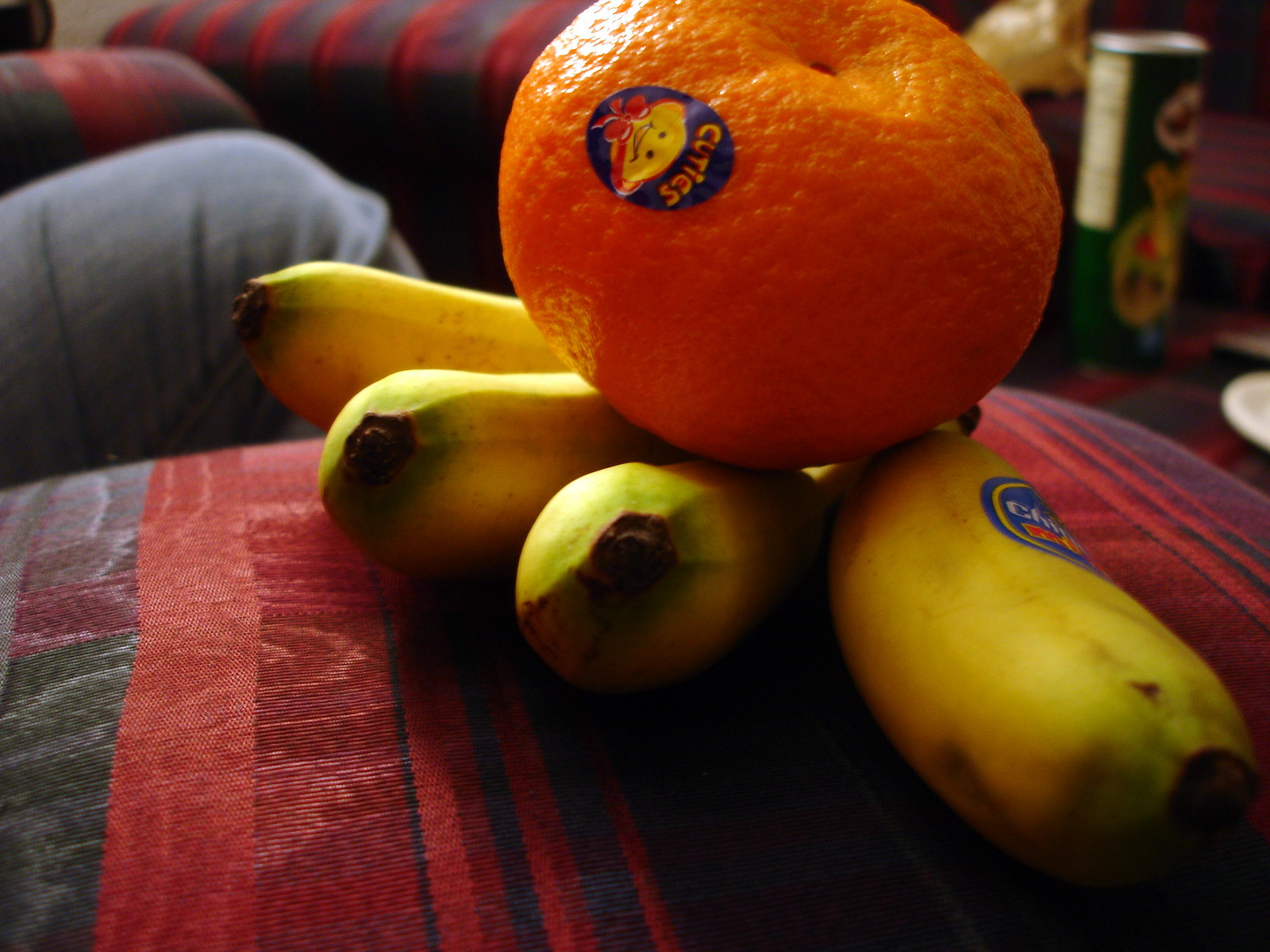This close-up photograph showcases an assortment of fruit, with the primary focal point being a mandarin orange positioned slightly off-center towards the upper part of the frame. The mandarin's sticker prominently features the brand "Cuties" along with a cheerful, cartoon-style lemon character sporting a bowtie. Beneath the mandarin orange, an arrangement of bananas extends outward, with one banana oriented towards the viewer in the lower right corner. A partially visible Chiquita sticker is present on the bananas. The fruits are placed on an armrest of a couch, distinguished by its vibrant orange-reddish color and accented with blue-green striped patterns. In the background, a person’s leg is noticeable, seated in the distance, and to the right side, an out-of-focus Pringles can is visible, although the flavor cannot be discerned.